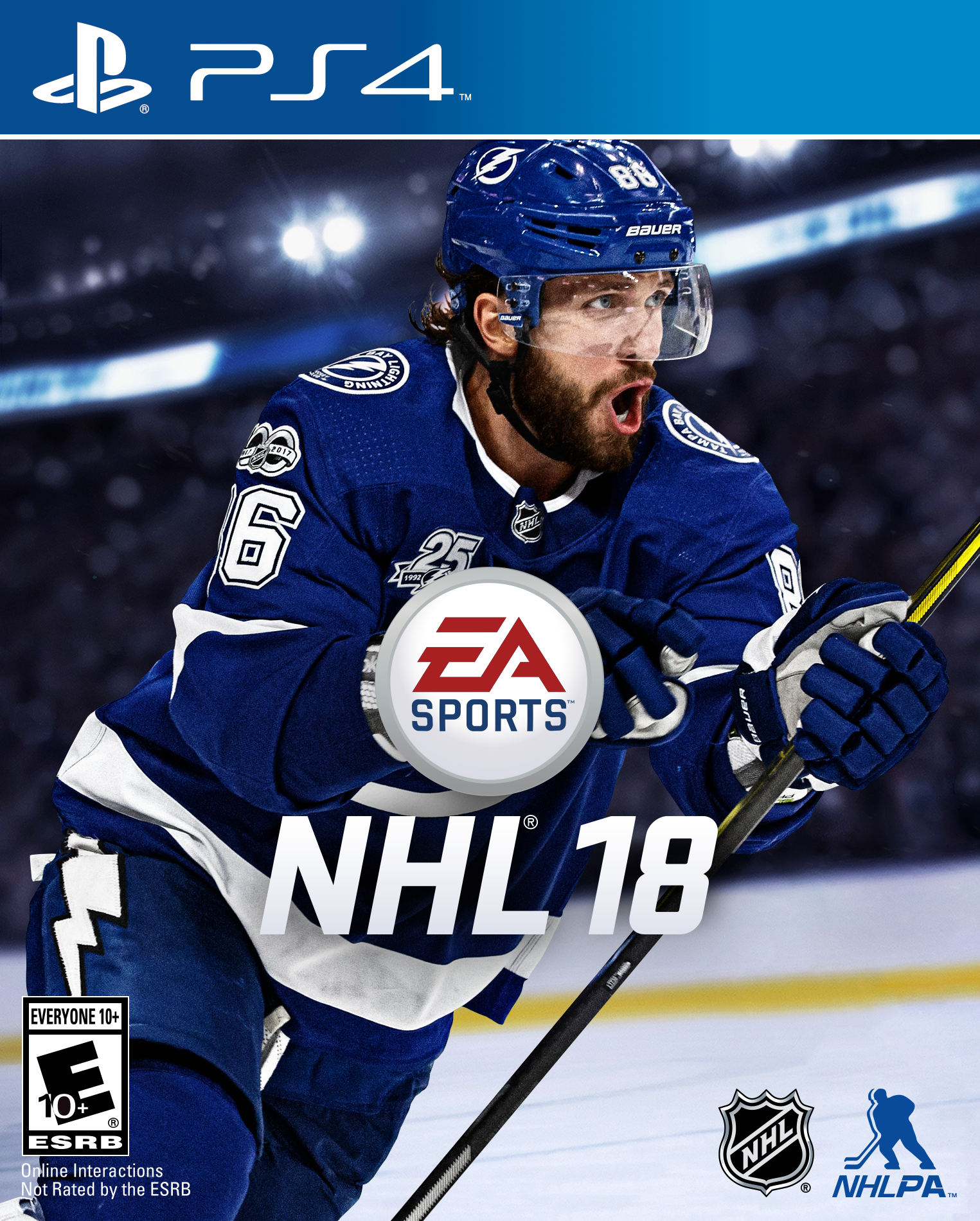This is an image of the cover for an NHL 18 PlayStation 4 (PS4) game. The top of the cover features the PS4 logo, displayed in white text within a blue rectangular background, accented by a white line underneath. Dominating the center of the cover is the iconic EA Sports logo, with "EA" in red and "Sports" in blue text inside a white circle outlined in gray. Below the logo, "NHL 18" is written in bold white text. 

The focal point of the image is a dynamic depiction of a hockey player mid-action, seemingly skating towards the right. He is fully clad in a blue uniform, including a blue helmet with a visor, blue gloves, and blue pants with a white belt. Distinctly visible on his uniform is the number "86" on his helmet and part of a number ending in "6" on his right arm. The player's outfit also features white socks and blue patches on the shoulders. His expressive face, boasting a beard and mustache, is visible with his mouth wide open, indicative of the intensity of the game. He clutches a hockey stick firmly in his hands.

In the background, blurred stands are visible, filled with enthusiastic fans, illuminated by glaring lights which add to the atmosphere of a live hockey game. The cover also includes the NHL logo in white on black in the lower right corner, along with the NHLPA logo, depicting a blue silhouette of a hockey player. The rating symbol of the disc is positioned in the left corner, completing the detailed cover design.